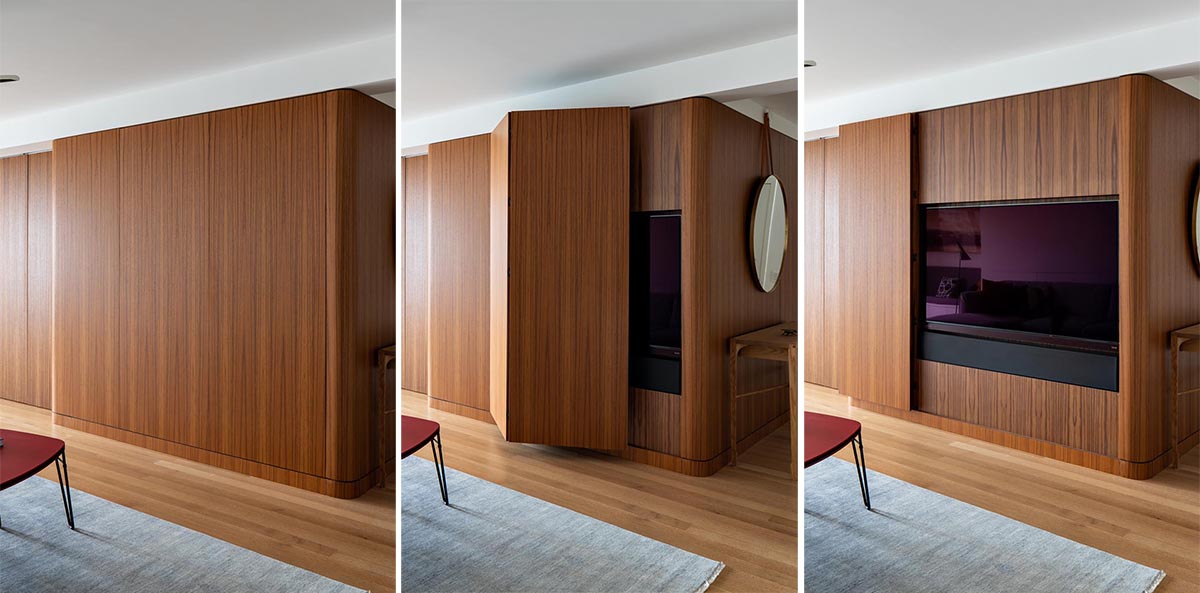A triptych of detailed indoor photographs showcases a modern living space featuring a red chair with metal legs positioned on a grey carpet over a brown hardwood floor in the lower left corner. The primary focus across all three images is a versatile wooden wardrobe situated against the backdrop of a wooden wall, advancing at an incline from the bottom right to the top left due to the camera’s perspective. 

In the first photo, the wardrobe is closed, presenting a seamless wooden facade. The second photo captures the wardrobe with its front door partially open, revealing a side mirror. In the final photo, the door is fully open, displaying a built-in, big screen TV, confirming its multifunctionality. The wooden tones of the wardrobe harmonize with the room's hardwood flooring, while the white ceiling and an exterior light source, possibly from a window, subtly illuminate the space.